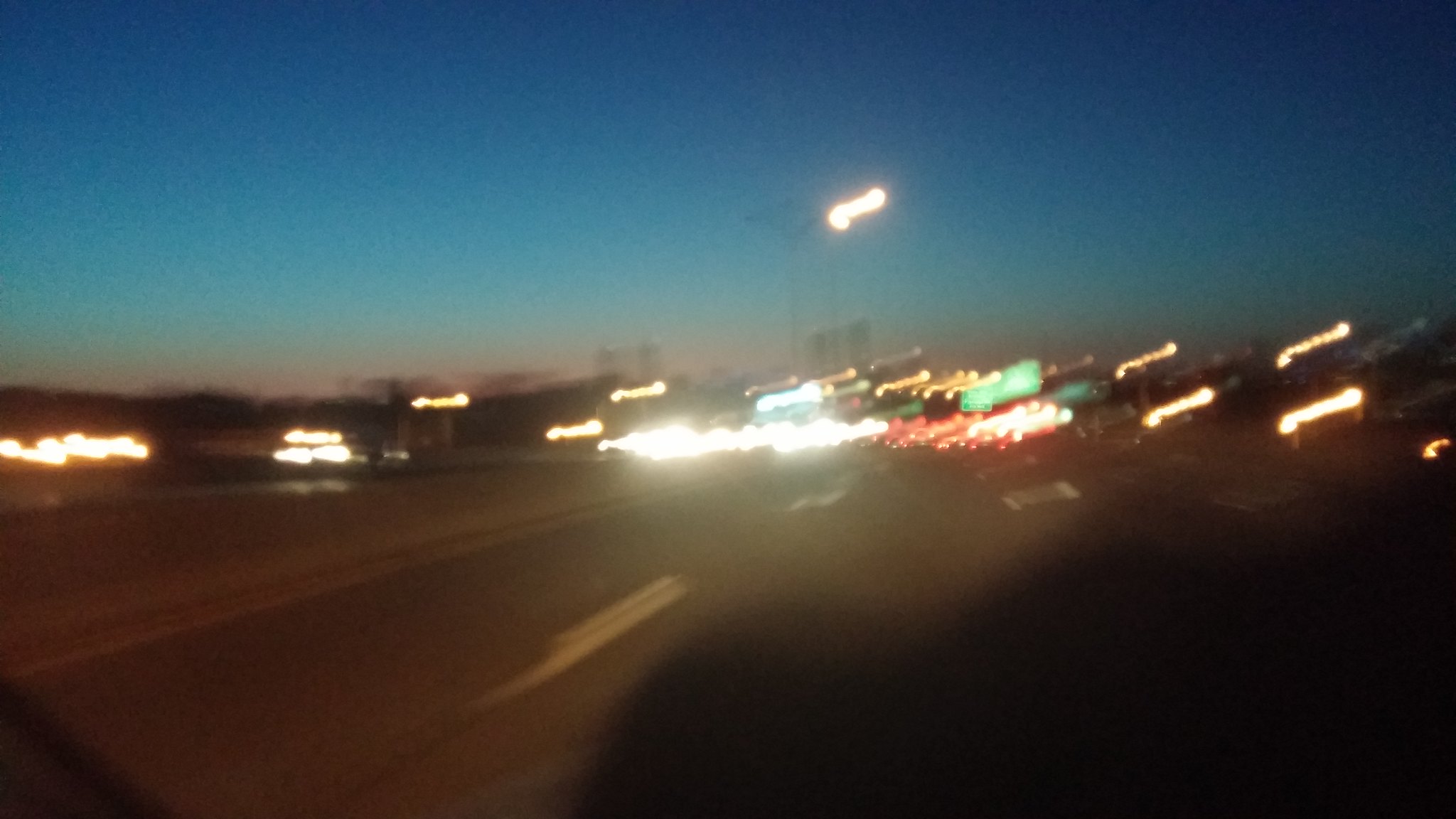This is a color photograph capturing a blurry roadside scene at dusk, imbued with motion blur that distorts fine details. In the foreground, a road stretches out, marked by broken lines, while towards the bottom left and extending to the bottom right corner, a dark shadow obscures part of the view. On the left, a pavement or possibly a strip of grass is faintly visible. The mid-section of the image is illuminated by a line of blurred lights, potentially car headlights or streetlights, arranged almost horizontally. Central to the composition, a series of street lights and power lines or poles rise into view. Above, the sky transitions from a reddish hue at the horizon to a light blue before deepening into a dark, almost navy blue towards the upper edges and corners, encapsulating the serene yet dynamic atmosphere of dusk.